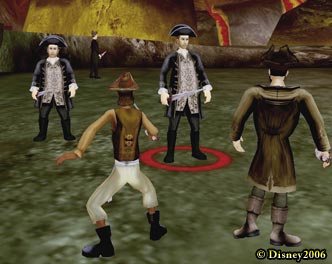The image is a detailed screenshot from a video game with an animation style that suggests a historical or adventurous theme. The scene features a large golden, red, and brown wall with a smaller brown wall at the base, situated on a green floor that gives the impression of a hilly landscape. The top right corner shows a hill, adding depth to the environment. 

Five characters are present in this scene. Two are facing the camera dressed in blue uniforms with grey shirts, blue jackets, and blue hats, possibly indicating a soldier or pilgrim-like attire. A red circle at the bottom highlights one of these figures. In contrast, two other characters – one in a cowboy hat and vest with white pants and dark cowboy boots, and another in a long coat with grey boots and an ornate hat, are seen from the back, suggesting a narrative or directional focus. 

The overall background includes a blue-grey sky with an indistinct cylindrical object in the upper left corner, hinting at a distant structure. In the bottom right corner, there is a watermark: "Copyright Disney 2006," establishing a timeframe and origin for the image.